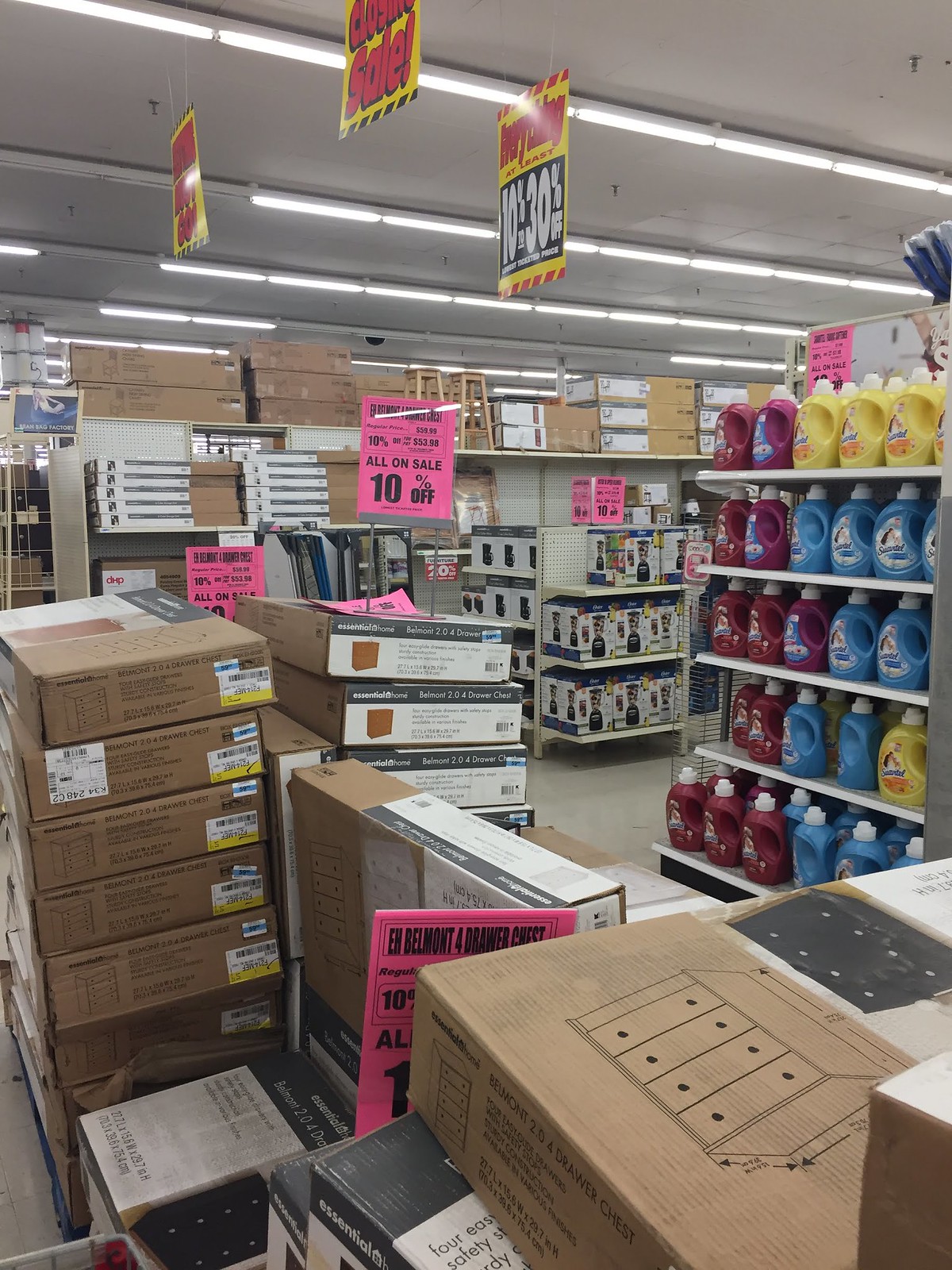The image portrays a melancholic scene inside a closing retail store. In the foreground, several boxed items are displayed for clearance, the nearest being a four-drawer bureau. The bureau features a pink sale sign, obscured as it leans against the box, indicating a discount but not revealing the exact percentage off. These pink signs are visible on various other items throughout the store. Suspended from the ceiling are prominently yellow, red, white, and black banners announcing the store's closure and current discounts, with the nearest sign noting a range of 10% to 30% off. The scene shows a section stocked with laundry detergent and fabric softener, with brightly colored red, yellow, and blue bottles orderly arranged on white shelves. The entire store is bathed in the stark, clinical light of fluorescent lamps, emphasizing the desolate atmosphere of the closing business.